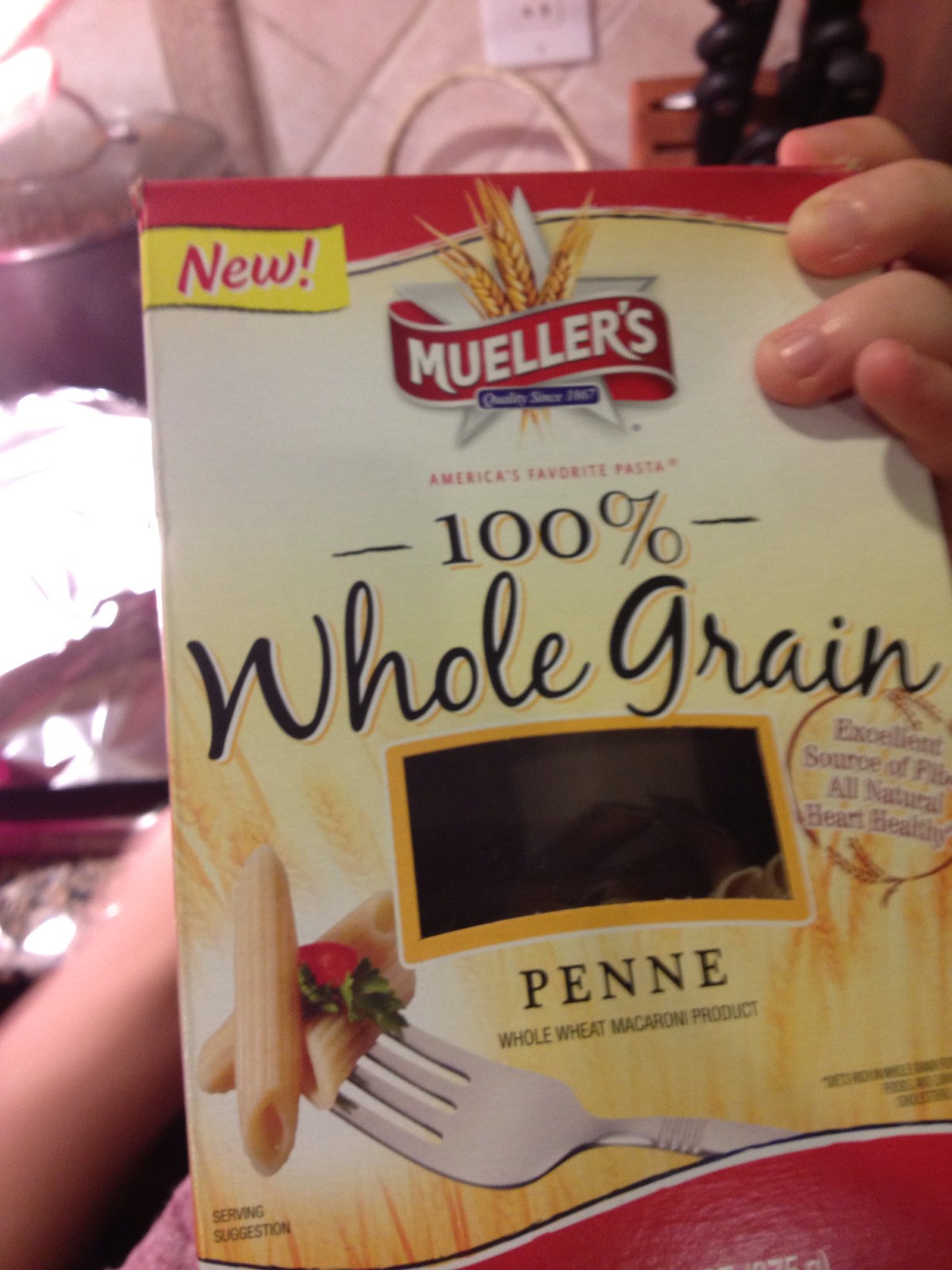The image features a box of penne pasta made from whole wheat. The box, constructed out of cardboard, displays a rectangular banner in the top left corner that announces "New." Directly to the right, a logo features the brand name "Mueller's" on a red ribbon wrapped around three large stalks of wheat. Below the logo, the text "America's Favorite Pasta™" is prominently displayed. Further down, the box describes the contents explicitly as "100% Whole Grain Penne Whole Wheat Macaroni Product." Additional highlights on the packaging emphasize that the pasta is an "Excellent Source of Fiber," "All Natural," and "Heart Healthy." The overall design and text aim to convey the wholesome and beneficial qualities of the product.